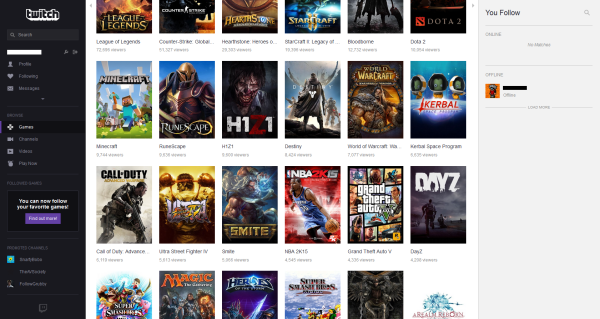Screenshot Description: 

The image is a detailed screenshot of the Twitch TV search menu interface. The backdrop is predominantly black, contrasted by white text on the left-hand side where various menu options are listed. These options include 'Profile,' 'Following,' and 'Messages.' Below these, there are additional categories such as 'Games,' 'Guides,' and 'Account.'

The central portion of the screenshot emphasizes searchable game titles. The interface includes a mix of colorful text in shades of pink and purple, aiming to highlight specific sections or important features. The listed games span an extensive range of popular titles, including:

- League of Legends
- Counter-Strike
- Hearthstone
- Starcraft: Legacy of the Void
- Bloodborne
- Dota 2
- Minecraft
- RuneScape
- H1Z1
- Destiny
- World of Warcraft
- Kerbal Space Program
- Call of Duty
- Street Fighter
- Ultra Street Fighter 4
- Smite
- NBA 2K15
- Grand Theft Auto V
- DayZ
- Super Smash Bros.
- Magic: The Gathering
- Heroes of the Storm
- Super Smash Bros. Melee
- Final Fantasy XIV: A Realm Reborn

To the right of the central game listing, there is another menu, used for managing follow statuses with distinct sections labeled for 'Online' and 'Offline' users. The 'Offline' section is highlighted with a unique avatar featuring a person with white hair and goggles. Directly beneath this menu, the name 'Lodemar' is displayed.

The entire interface is crafted for ease of navigation, allowing users to quickly locate and access their favorite games and streamers.